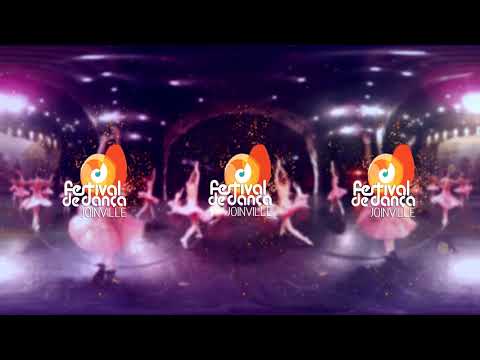The advertising poster features a striking triptych design against a predominantly black background. In the center, the backdrop is subtly illuminated with a hint of purple, creating a sparkly and translucent effect, augmented by light reflections on either side. The focal point of the poster is the three mirrored logos aligned horizontally across the middle. Each logo comprises an orange circle with what appears to be a wing-like or orange slice-shaped element on the side. Within the circle, there is a unique white symbol with a blue center, resembling a stylized music note.

Beneath each logo, the text "Festival de Danza" is prominently displayed in bold, white bubble letters, followed by "Joinville" in a slimmer, basic white font. The background imagery includes a blurred depiction of ballerina dancers, creating a sense of motion as they twirl in a circle. These dancers, numbering between five to fifteen, are dressed primarily in white and appear to be performing in a dance hall, complete with soft lighting that enhances the overall ethereal atmosphere. Thick black borders at the top and bottom of the image frame the poster, adding to its striking visual appeal.